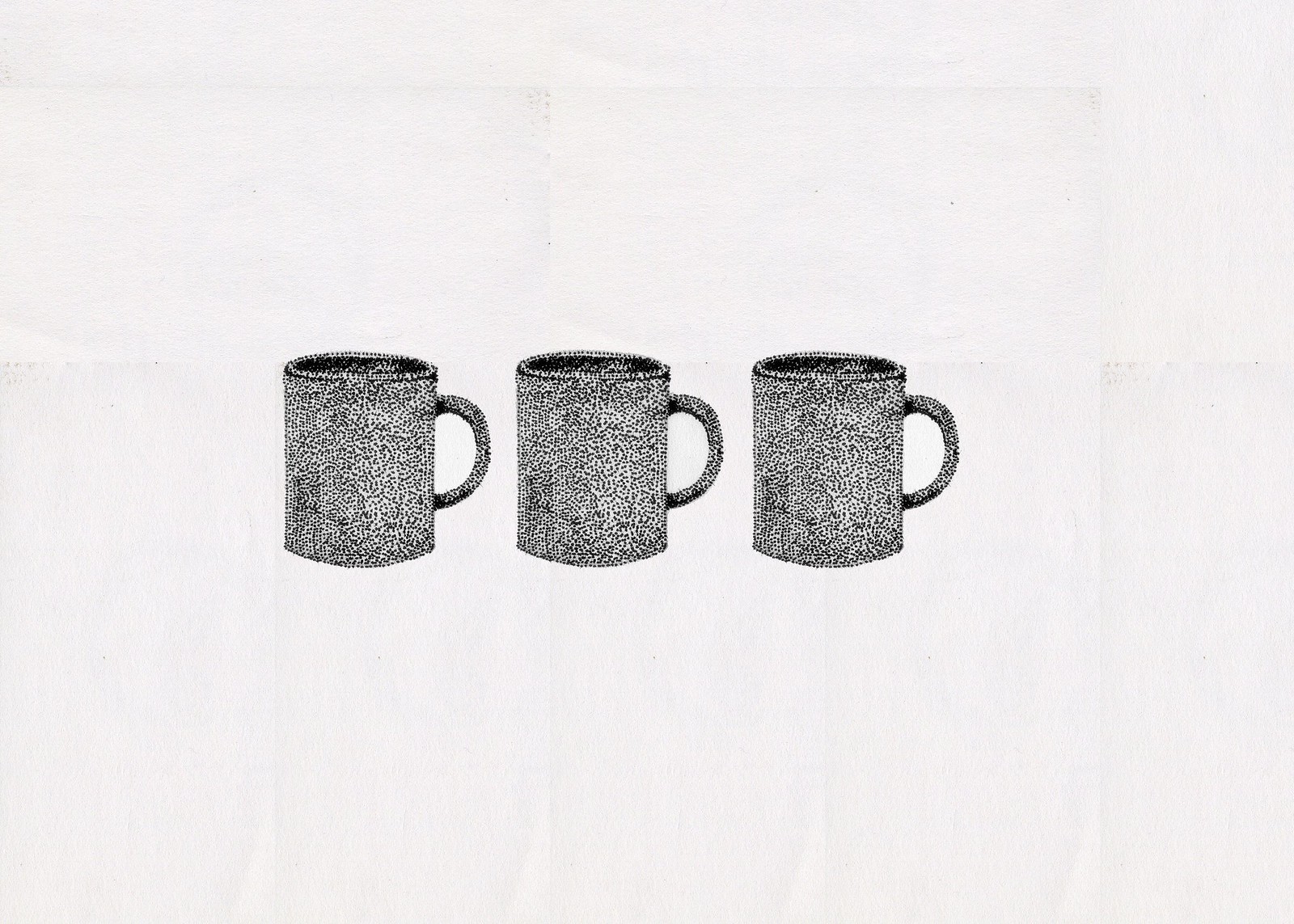This image depicts a meticulously drawn lineup of three identical mugs, rendered in black ink on a faintly textured white sheet of paper, which is set against a white background or tabletop. The mugs are arranged side by side in a row, with each handle protruding to the right, forming a subtle semicircle. The style of the drawing showcases pointillism, where the mugs are fashioned out of densely clustered black dots that cover their entire surface, including the handles and inner rims. This speckled shading technique provides a textured appearance and makes the inner rims appear darker, almost grey. Upon closer inspection, the intricate pattern of dots might even create an impression of a lion's face within the mug's surface, adding a layer of visual intrigue to the otherwise simple black-and-white illustration.